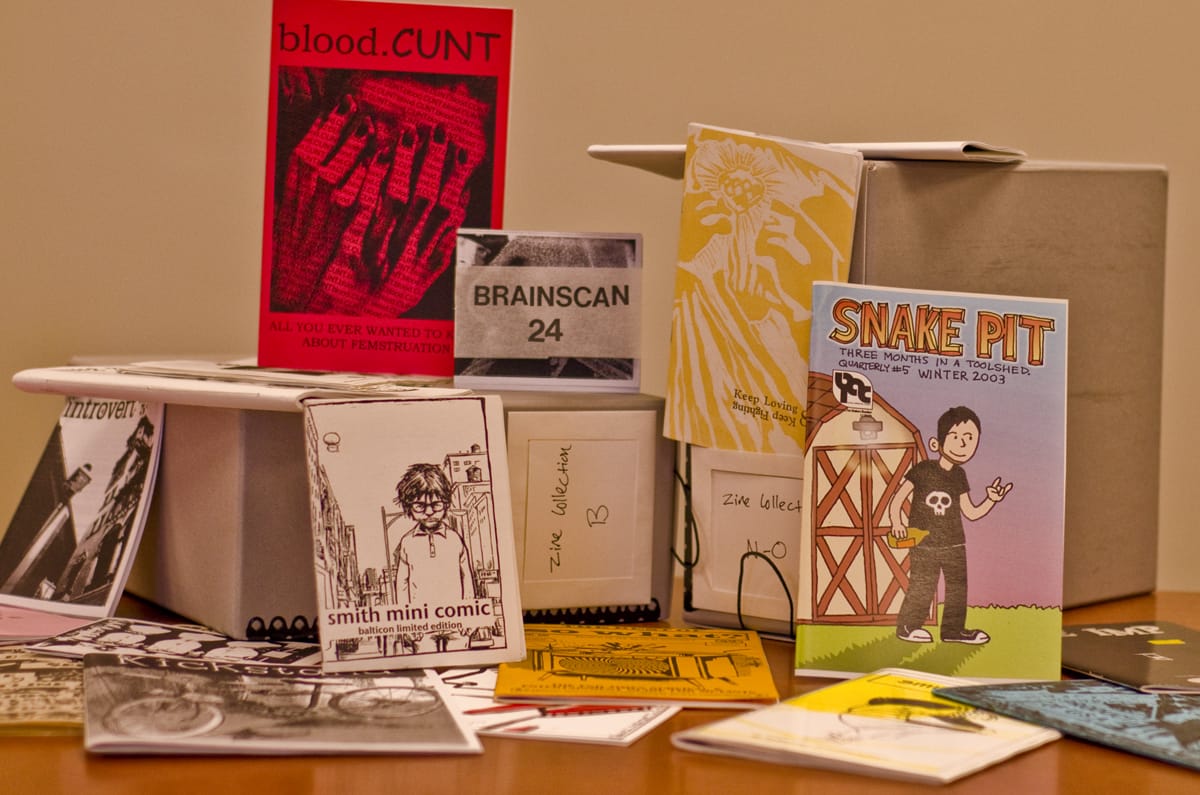This image displays an array of various small books and comic booklets, predominantly set against a brownish backdrop, giving the entire scene a sepia-toned hue. Arranged both laying flat and standing upright near cardboard boxes on a wooden table, the collection includes distinct titles such as "Snake Pit," a book featuring a young man holding a bottle and making a devil's horn gesture in front of a stylized toolshed titled "Three Months in a Toolshed, Quarterly, Winter 2003." Central to the display is a black and white booklet named "Smith Mini Comic," depicting a scowling man, and another similarly monochromatic leaflet titled "Brainscan 24." Among the vibrant covers, a striking red book titled "Blood Cunt" stands out, contributing to the diverse and unique assortment of graphic novels and mini-comics showcased in this brown-hued exhibition.